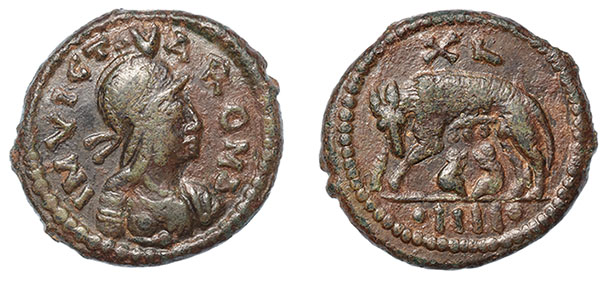The image features two ancient, bronze-colored coins with a slightly reddish hue, set against a plain white background. These coins appear worn and rustic, suggesting their age and historical significance. The left coin displays a roughly engraved image of a man, possibly a soldier, wearing what seems to be a hat. Around the portrait are letters forming "INVICTVAROM," presumably from a Latin inscription. The right coin showcases an animal, likely a wolf or dog, accompanied by additional Latin characters. This coin also features a pattern of small circles along the edge. Both coins have rugged edges and a scalloped border, giving them an artifact-like appearance. It's unclear whether these images represent two sides of the same coin or two separate coins.